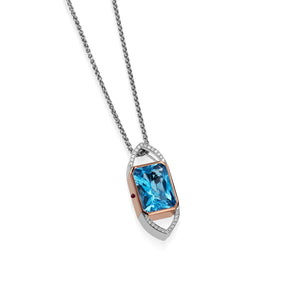This image features a necklace presented against a white background, focusing on the pendant. The necklace has a silver chain that runs diagonally from the upper left to the lower right. The pendant is medallion-shaped, resembling a wide oval with pointed ends, somewhat akin to a squashed football.

The main highlight of the pendant is a large, vertically-oriented rectangular gem, predominantly blue with hints of black. The gem appears to be cut and polished, housed within a rose gold or copper frame that accentuates its shape. This frame is encased in another layer of silver, forming an arch at both the top and bottom of the gem. This second layer is detailed with tiny, clear stones, possibly diamonds, embedded along the edges, adding a touch of sparkle to the piece.

While the image is small and of poor resolution, these intricate details can still be discerned, showcasing the elegance and complexity of the necklace's design.